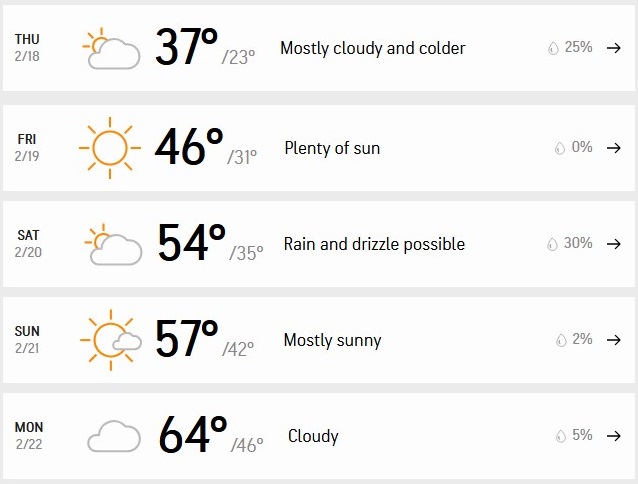This image appears to be a screenshot of a weather forecast, likely from a tablet or desktop, given its wide dimensions. The forecast covers a five-day period, but unfortunately, the location is unspecified, with no mention of city, state, or country.

**Five-Day Weather Forecast:**

- **Thursday, February 18th:** 
  - **Weather:** Mostly cloudy 
  - **Temperature:** High of 37°F, Low of 23°F
  - **Precipitation:** 25% chance
  
  A small pictogram depicts the sun partially obscured by clouds, indicating colder and mostly cloudy conditions.

- **Friday, February 19th:**
  - **Weather:** Plenty of sun
  - **Temperature:** High of 46°F, Low of 31°F
  - **Precipitation:** 0% chance

  The forecast shows a bright sun, suggesting a clear and sunny day with no expected precipitation.

- **Saturday, February 20th:**
  - **Weather:** Mostly cloudy with rain possible
  - **Temperature:** High of 54°F, Low of 35°F
  - **Precipitation:** 30% chance

  An icon of the sun largely hidden by clouds points to potential rain and drizzle.

- **Sunday, February 21st:**
  - **Weather:** Mostly sunny
  - **Temperature:** High of 57°F, Low of 42°F
  - **Precipitation:** 2% chance

  A pictogram shows a tiny cloud in front of the sun, indicating a predominantly sunny day.

- **Monday, February 22nd:**
  - **Weather:** Cloudy
  - **Temperature:** High of 64°F, Low of 46°F
  - **Precipitation:** 5% chance
  
  The day is forecast to be cloudy, as denoted by the icon of a single cloud.

The layout suggests interactive elements such as arrows to possibly access more detailed forecasts, but these features are not fully visible in the image provided.